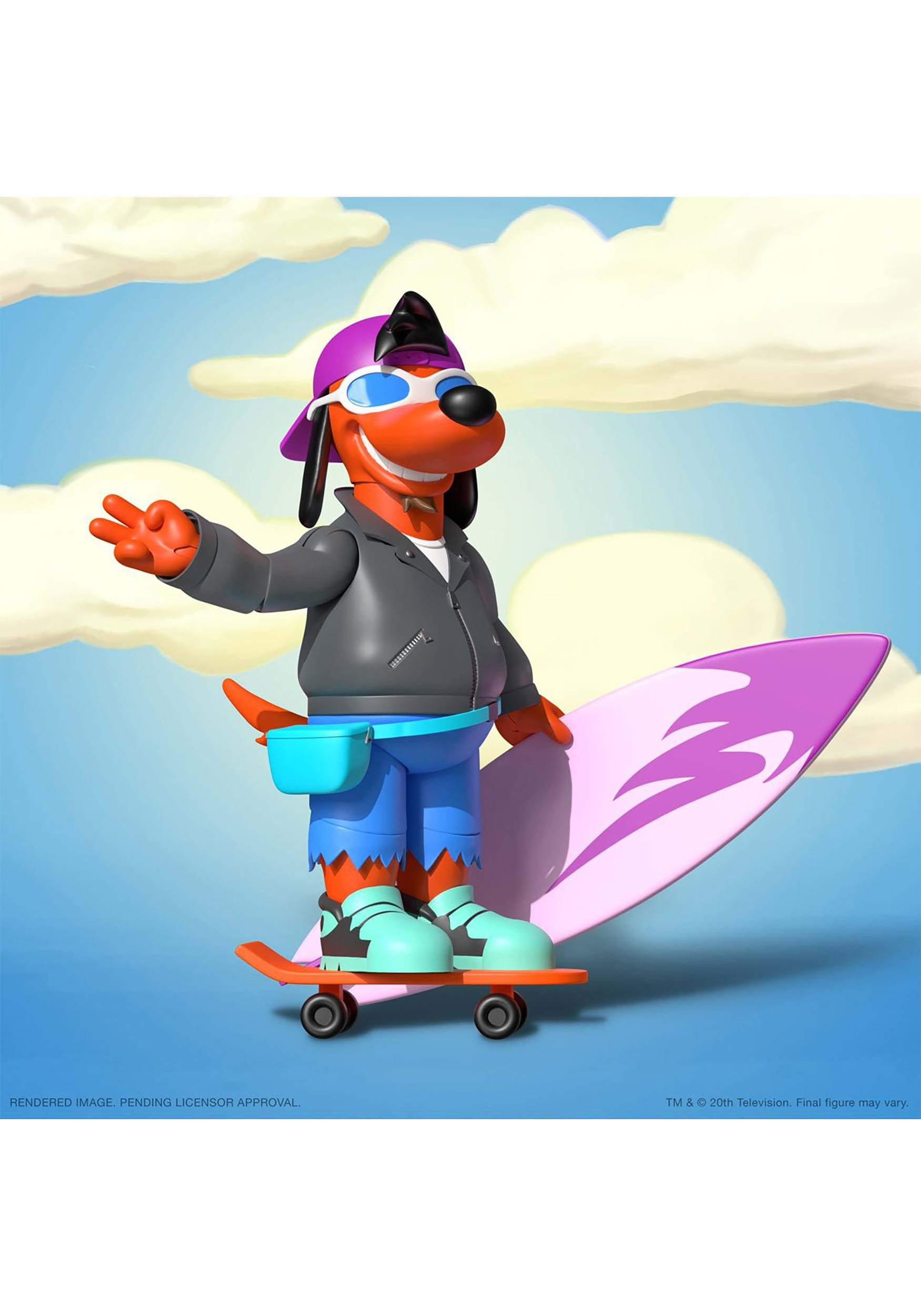This image depicts a vibrant CGI cartoon scene featuring an anthropomorphic, orange dog adorned in an eclectic mix of human clothing and accessories, all set against a blue sky dotted with white and tinged-yellow clouds. The charismatic canine sports a backwards purple baseball cap, blue sunglasses with white frames, a leather jacket over a white t-shirt, and a light blue fanny pack strapped around his waist. His outfit is completed with cut-off, torn blue jeans and mismatched sneakers—black and light blue in one rendition, green and brown in another. The dog, striking a playful pose with a peace sign, stands confidently on an orange skateboard with black wheels. Clutched in his left hand is a dual-toned surfboard, primarily purple with lighter purple or pink accents, adding to his adventurous and quirky look.